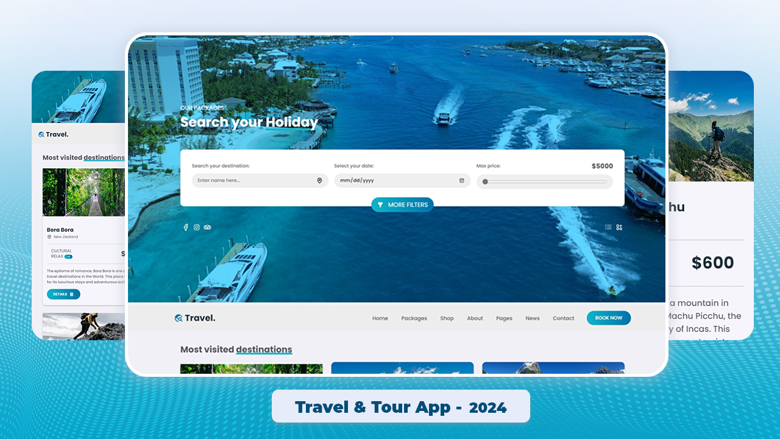The image features three posters, with the central one being the largest and flanked by two smaller ones on either side. Dominating the middle of the graphic is the text "Search Your Holiday" in white. Beneath this, within a rectangular section, there are three input fields: "Search Your Destination," "Search or Select Your Date," and "Min Price." Each field has a corresponding input area: "Search Your Destination" prompts users to "Enter name here," "Search or Select Your Date" displays a placeholder formatted as "MM/DD/YYYY," and "Min Price" features a scroll bar allowing users to adjust the value.

The backdrop of the image showcases a vast expanse of water, dotted with several boats. In the top left corner, a large white building stands prominently. At the bottom center, the words "Travel and Tour App 2024" appear on a grayish background. 

To the far right of the image, partially cut off, a person is depicted standing on a mountain, with a price tag of "$600" visible at the bottom of this section.